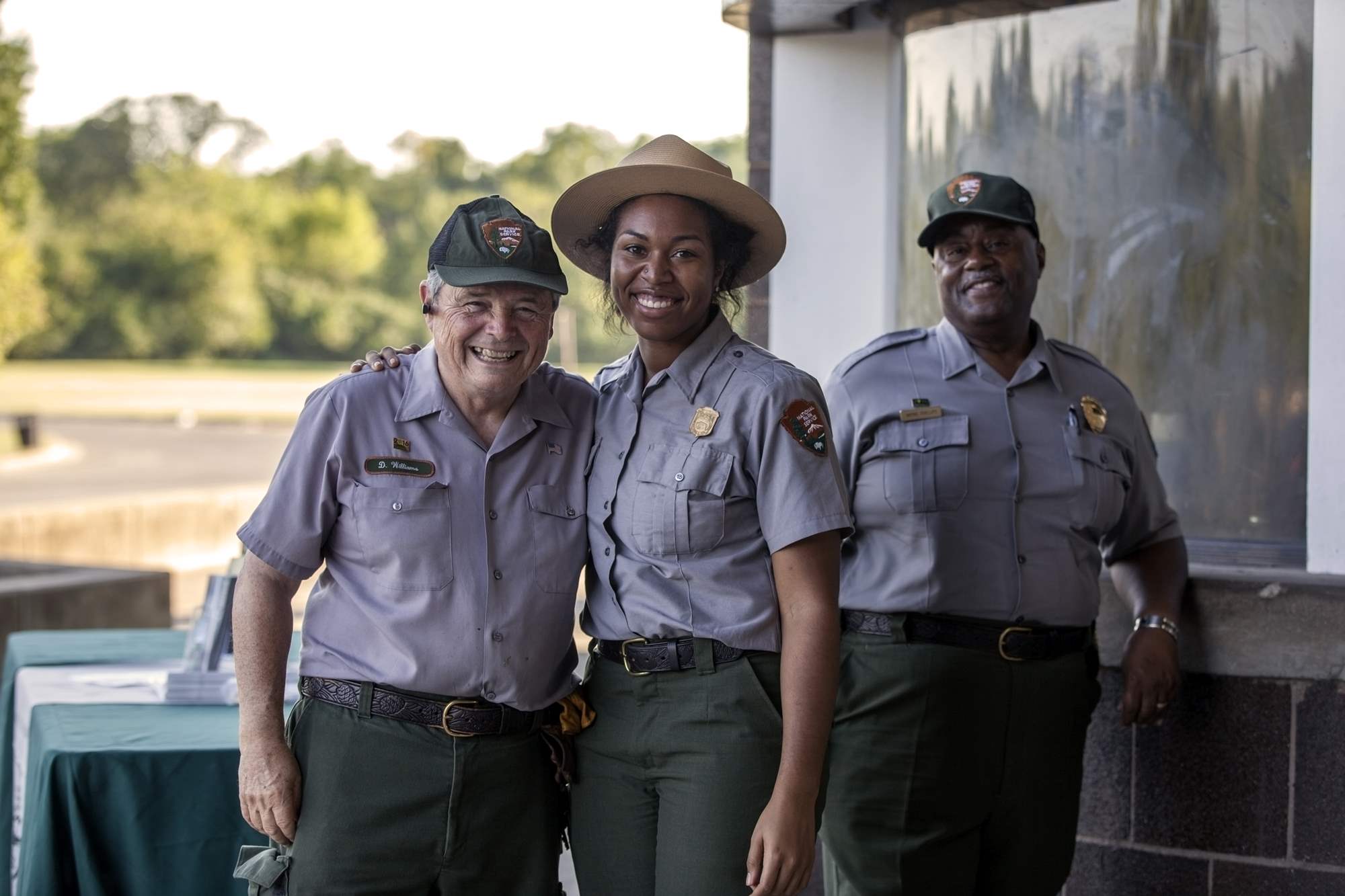This photograph, taken outdoors during the daytime with clear, natural lighting, showcases three uniformed park rangers posing together. Each ranger is dressed in a short-sleeve, button-up blue shirt adorned with a name tag on one side and a badge on the other, complemented by a patch on the shoulder. They wear black belts and forest green pants. The ranger on the left is an older white man sporting a green hat with an insignia patch and smiling warmly with squinted eyes and an open-mouthed grin. Standing in the middle is a younger black woman, her arm affectionately around the older man. She wears a tan brimmed hat and smiles brightly, her hair hidden under her hat. Slightly behind them on the right is a middle-aged black man wearing a similar green hat as the older man. He has a hint of a beard and stands slightly back with a composed expression. The background features a table covered with a green tablecloth, a gray cinder block building with a window, a field, a road, and distant trees, adding a touch of natural and rustic scenery to the setting.